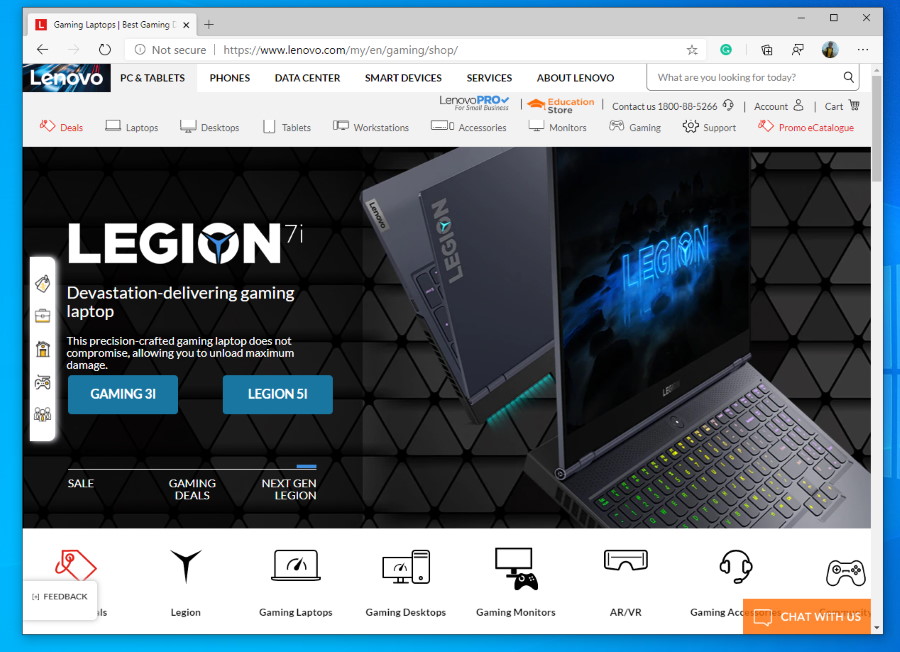This image is a detailed screenshot of a computer browser displaying a webpage titled "Gaming Laptops - Best Gaming." The top left corner of the browser shows a tab named "Gaming Laptops, Best Gaming," followed by a close button (X), and a plus sign for adding a new tab. On the top right corner, the standard minimize, maximize, and close buttons are visible.

Below the browser tabs, there is a navigation bar containing a back arrow icon and an address bar next to it, followed by several unidentified icons on the right. Directly beneath this is a series of clickable tabs, including "Lenovo," "PC and Tablets," "Phones," "Data Center," "Smart Devices," "Services," "About Lenovo," and a search bar. Further below, on the right side, there is contact information reading "Lenovo Pro Education Store, contact us at 1-800-88-5266," alongside account management and shopping cart icons.

Spanning the width of the page is a navigation menu with options for "Deals," "Laptops," "Desktops," "Tablets," "Workstations," "Accessories," "Monitors," "Gaming," "Support," and "Promo and Catalog." The main focus of the screenshot is an image of a Lenovo laptop. To the left of the laptop, there are clickable options labeled "Gaming 31" and "Legion 51." At the bottom of the main image, various links are listed, including "Deals," "Legion," "Gaming Laptops," "Gaming Desktops," "Gaming Monitors," "AR/VR," and "Gaming Accessories." An opaque orange "Chat with us" button pops up from the bottom right corner, inviting users to initiate a live chat.